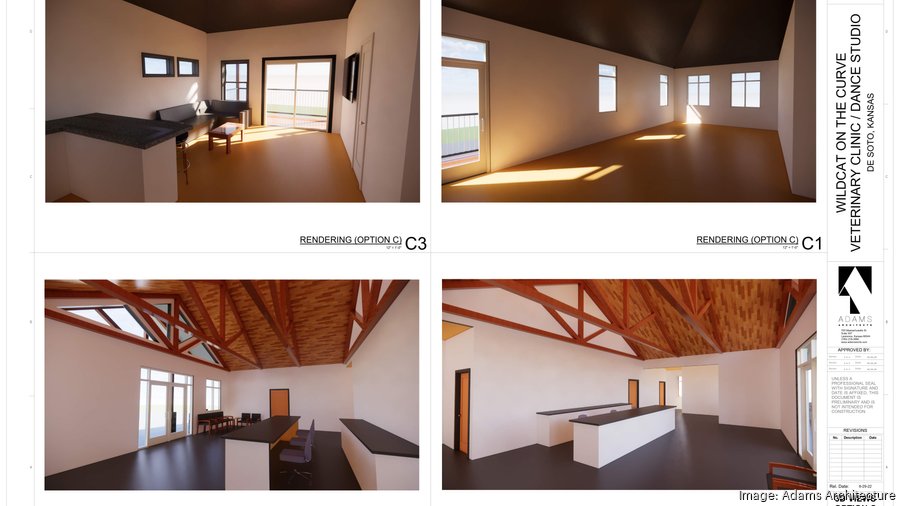The composite image showcases four renderings of an office-type space labeled "Wildcat on the Curve Veterinarian Clinic and Dance Studio." 

In the upper left corner (labeled C3), the rendering features a cozy area with a black countertop island and a sofa and love seat set around a small coffee table. Large windows allow natural light to flood the space, which also includes a door leading out to a patio. 

The upper right image (labeled C1) depicts a bright, empty room with five windows letting in sunlight, creating a well-lit atmosphere. This room has a hardwood floor and a door on the left-hand side, with white walls and a vaulted wooden ceiling.

In the bottom left, we see a reception area with a black marble-topped counter and two office chairs. Behind this is another counter, similarly black-topped, with windows and a vaulted ceiling with exposed wood beams, creating a dynamic architectural feature. The floor is a deep black, which contrasts with the white walls.

The bottom right image mirrors the adjacent reception area with another black countertop and chairs positioned in front and behind it. The space includes doors leading to other areas, with consistent elements of a black floor, white walls, and a vaulted wooden ceiling.